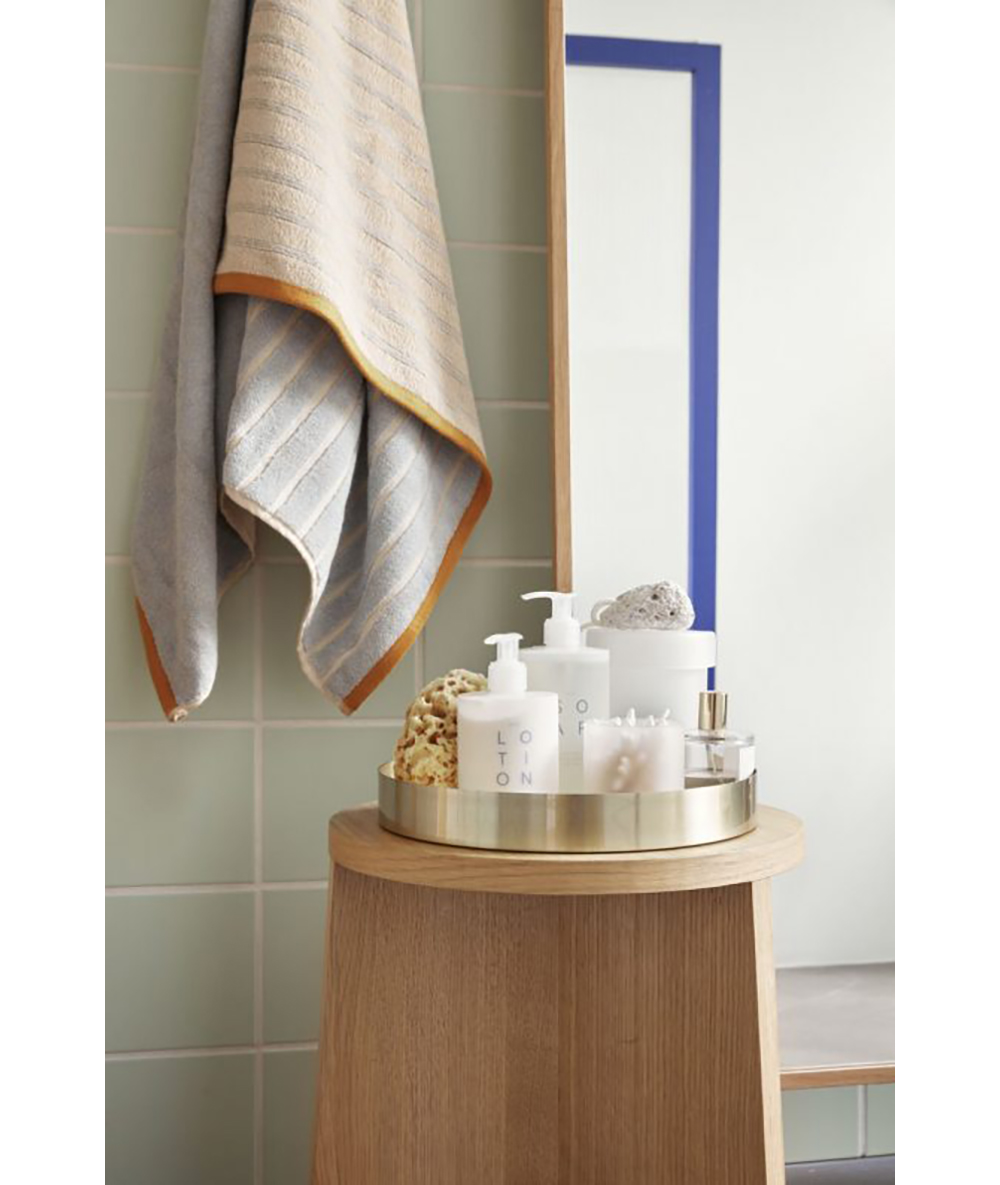The photograph captures a serene bathroom scene with meticulous detail. On the left side, a light gray tiled wall is visible, with light beige grout filling the gaps between the tiles. From the top of this wall, a towel is elegantly draped. The towel features an exterior design of beige with light gray horizontal lines and is bordered by a gold strip at the edge. The inside of the towel, visible due to its hanging position, reveals a very pale blue color adorned with white lines.

Running along the edge of the tile wall on the right side is a strip of natural wood molding, providing a subtle yet charming contrast. The right side of the photograph showcases a pristine white wall. Near the top, the corner of a blue rectangle, likely the frame of a mirror, peeks into the frame.

At the center of the scene, a round wooden table stands with an inviting presence. The table is supported by rectangular wooden legs that converge in the center, giving it a sturdy yet stylish appearance. Placed at the heart of the tabletop is a circular silver-rimmed plate, neatly organized with various bath items. The plate holds two white bottles with pumps—one slightly larger than the other—a beige loofah sponge, and a white candle, completing the tranquil and orderly ambiance of the bathroom.